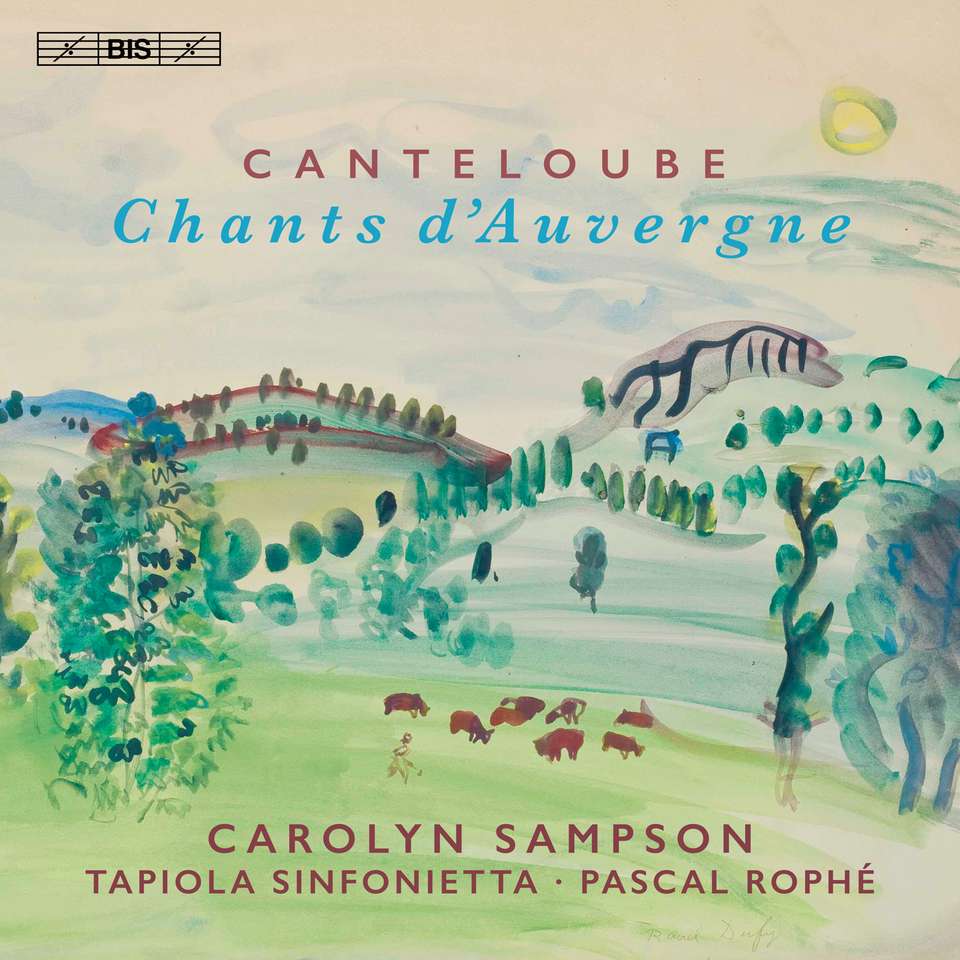The image features a quaint watercolor painting of a pastoral countryside, possibly an album cover. In the forefront of the painting, a shepherd with a rake or hoe stands among grazing brown cows on a lush green pasture. The landscape extends into rolling hills dotted with various blue and green trees, accented by occasional red and purple hues on the mountains and foliage. A pale sky with light clouds rests above the scene. Written across the top of the image in elegant fonts are the words "Cantaloupe Chants d'Auvergne" by Carolyn Sampson, accompanied by the "Tapiola Sinfonietta" and "Pascal Roffé." Additionally, there are musical notations and the acronym "BIS" in the top left corner, adding a whimsical, melodic touch to the overall composition.